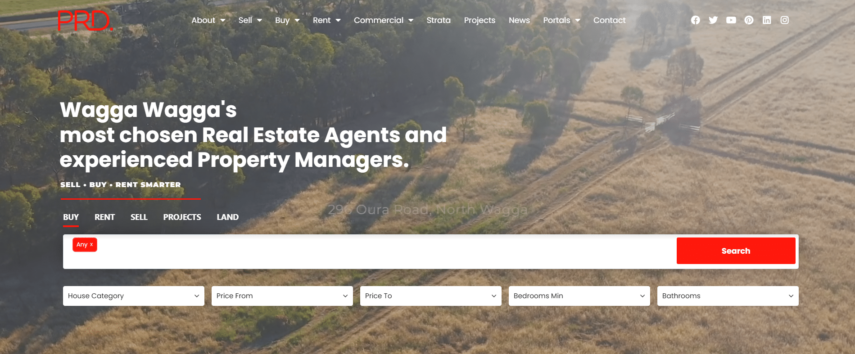This image is a cropped screenshot featuring the header of the PRD website, a company specializing in real estate and property management. The background is an aerial view showcasing expansive rural land dotted with trees. Prominently displayed in the center toward the left-hand side is a headline that reads, "Wagga Wagga's Most Chosen Real Estate Agents and Experienced Property Managers," in bold white text. Beneath this headline, in much smaller white letters, the slogan "Sell, Buy, Rent, Smarter" is visible, followed by a thin red line.

The header also includes a navigation bar listing five categories: Buy, Rent, Sale, Projects, and Land. The 'Buy' category is selected, highlighted by a red underline. Dominating the header is a large search box that spans the entire width of the page, with a prominent red 'Search' button on the right-hand side. Below the search bar are five drop-down boxes neatly aligned in the center. These boxes are labeled: House Category, Price From, Price To, Bedrooms Minimum, and Bathrooms. The rest of the webpage is not visible in this cropped screenshot.